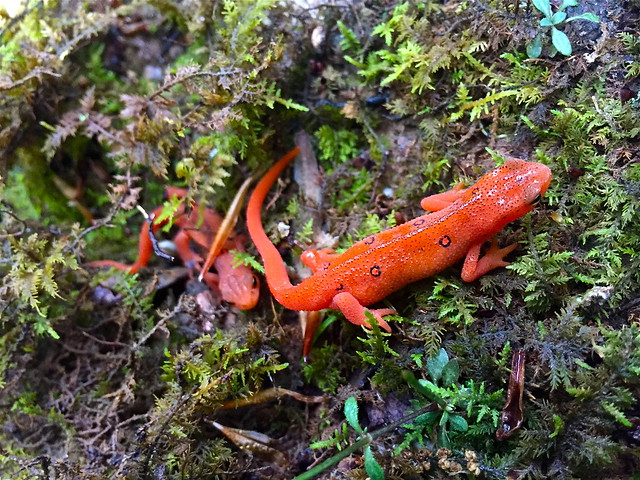This detailed photograph captures a pair of vibrant orange salamanders, speckled with intricate black patterns and hollow black circles lining their spines. The salamanders, which closely resemble newts with smooth, damp, and shiny skin, are crawling across a damp, moss and lichen-covered earth, surrounded by small green ferns and leafy plants. The larger salamander, positioned on the right, is climbing upwards with its tail curved upwards perpendicular to its body, and a faint white line extends down its back from its head to where its tail begins. This line is flanked by three or four outlined black dots. The second, smaller salamander follows behind, partially obscured by foliage and positioned further away, with its tail pointing out to the left. The ground glistens with moisture, enhancing the vivid colors and details of these captivating creatures.